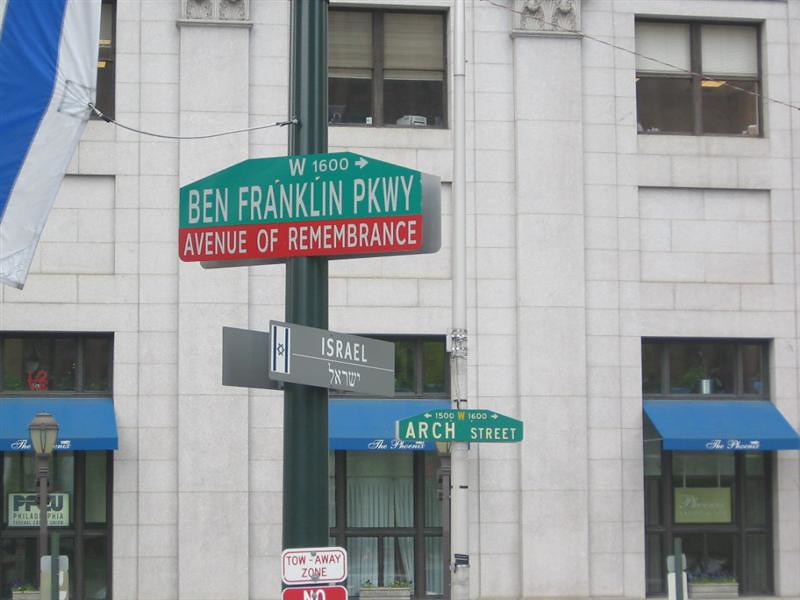The image depicts a white modern brick building with two rows of three windows each. Blue awnings with white lettering, possibly indicating businesses, adorn the ground floor windows. Prominently featured in the foreground is a green metal pole adorned with multiple signs. At the top, a green sign with white font reads "Ben Franklin Parkway," followed by a red sign with white lettering stating "Avenue of Remembrance." Below these, a gray sign with the word "Israel" and a vertically oriented Israeli flag is visible. Just beneath this, "Arch Street" is displayed on a green background. Additional signs on the pole indicate a tow-away zone with no parking. The scene, devoid of visible street pavement but filled with various signs, strongly suggests an urban setting.